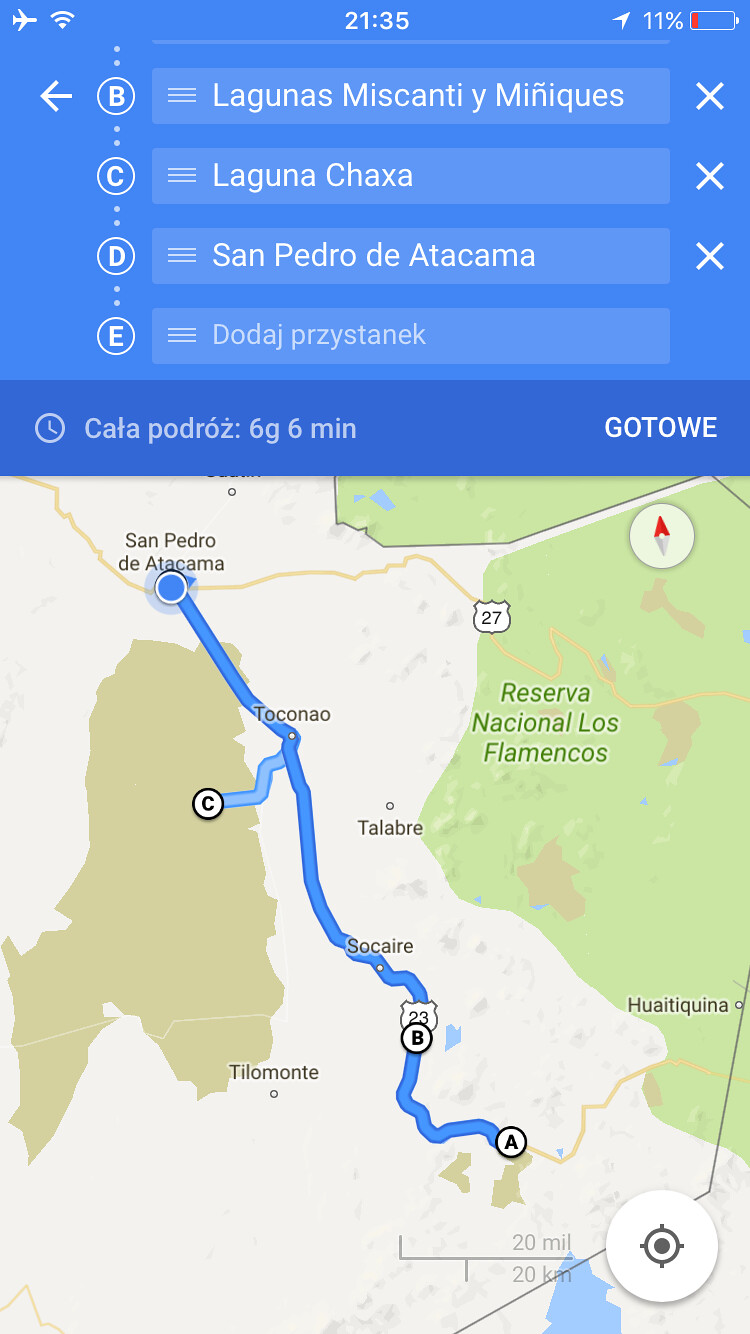The image appears to be a screenshot from a navigation or mapping application on a smartphone. At the top of the screen, several destinations are listed in Spanish, denoted by the letters B, C, D, and E. The locations include "B: Lagunas Miscantiae Benignas," "C: Laguna Chocsa," "D: San Pedro de Atacama," and "E: Dodage Briztanic." Below this list, the map portion of the app is visible, featuring a highlighted route in blue that connects these destinations. The map itself displays various terrain features, with sections of white and green representing different land types, and small blue areas indicating bodies of water.